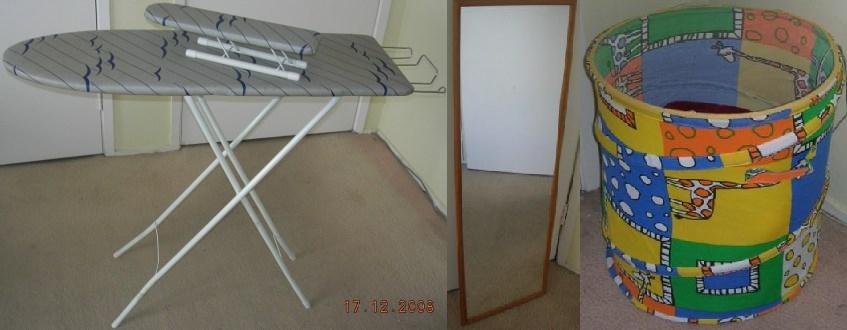The image is a rectangular photo collage made up of two square photos placed side-by-side. The left photo displays a large ironing board covered in gray fabric featuring angled lines and blue birds in flight. It stands on long, criss-crossing white legs. On top of this ironing board sits a much smaller ironing board, presumably for ironing smaller items like socks, sleeves, or pant legs. This mini ironing board also has white legs designed to stand on surfaces. In the bottom right corner of this image, there is a timestamp indicating the date "17 12 2003," which suggests the photo was taken with a point-and-shoot camera. The background reveals white doors separated by a cream-colored wall section and light brown carpet underneath.

The right photo captures a full-length mirror with a brown wooden frame. Positioned next to the mirror is a round toy basket featuring a colorful design with shades of yellow, blue, green, orange, and white, and adorned with images of a giraffe, zebra-like patterns, and clouds against a blue sky. This vibrant toy basket rests on a gray floor.